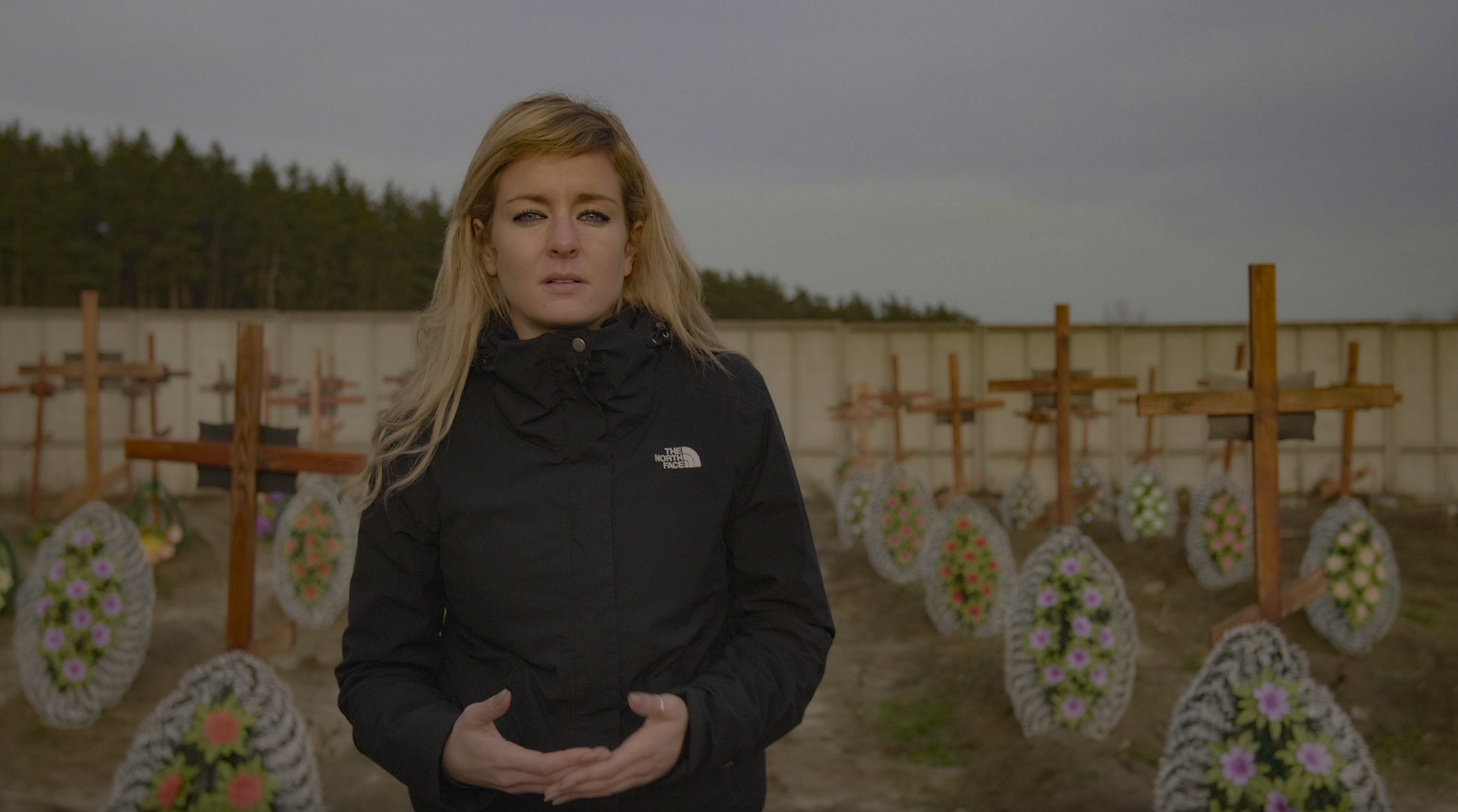The image depicts a solemn white woman with blonde hair and colored eyes, standing in what appears to be a makeshift graveyard. Her hair is fairly long, and she is donning a black North Face jacket with the logo visible on the left side of her chest. She stands amidst numerous grave markers, each marked by a simple wooden cross. Beside each cross is an egg-shaped flower arrangement or bouquet. Her hands are clasped together in front of her waist, and she has a somber expression as she faces the viewer. Behind her, a tall fence sections off the area, with a dense forest visible in the background. The sky is overcast, adding to the dismal mood of the scene. The entire image evokes a sense of solemnity and respect, possibly indicating that this is a memorial or a recently established graveyard.